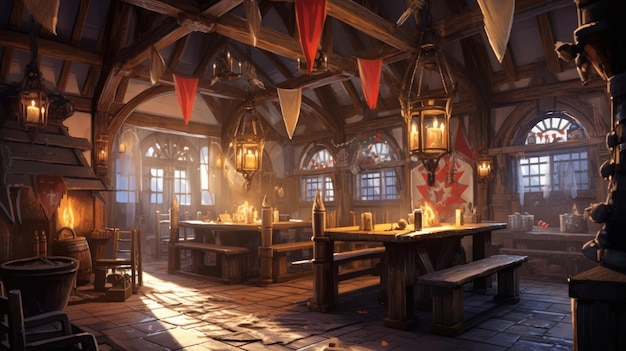This sketch depicts the interior of a medieval-style tavern, reminiscent of 14th or 15th-century England. The stone floor supports a variety of heavy wooden tables and benches, some of which are set with glasses and utensils. Detailed woodworking adorns the sides of the columns, adding to the rustic ambiance. The ceiling is crisscrossed with sturdy wooden beams from which red and off-white triangular pennants hang. Several glass chandeliers, each holding multiple lit candles, provide a warm, flickering light to the otherwise dim room. In the center left, a crackling yellow and orange fire burns in a stone fireplace, above which additional candles are lit. Flanking the fireplace, there's a wooden barrel and a couple of chairs, including a rocking chair. Light streams softly through the arched windows, casting a dusty glow across the room, highlighting the intricate details and historical charm of the scene.